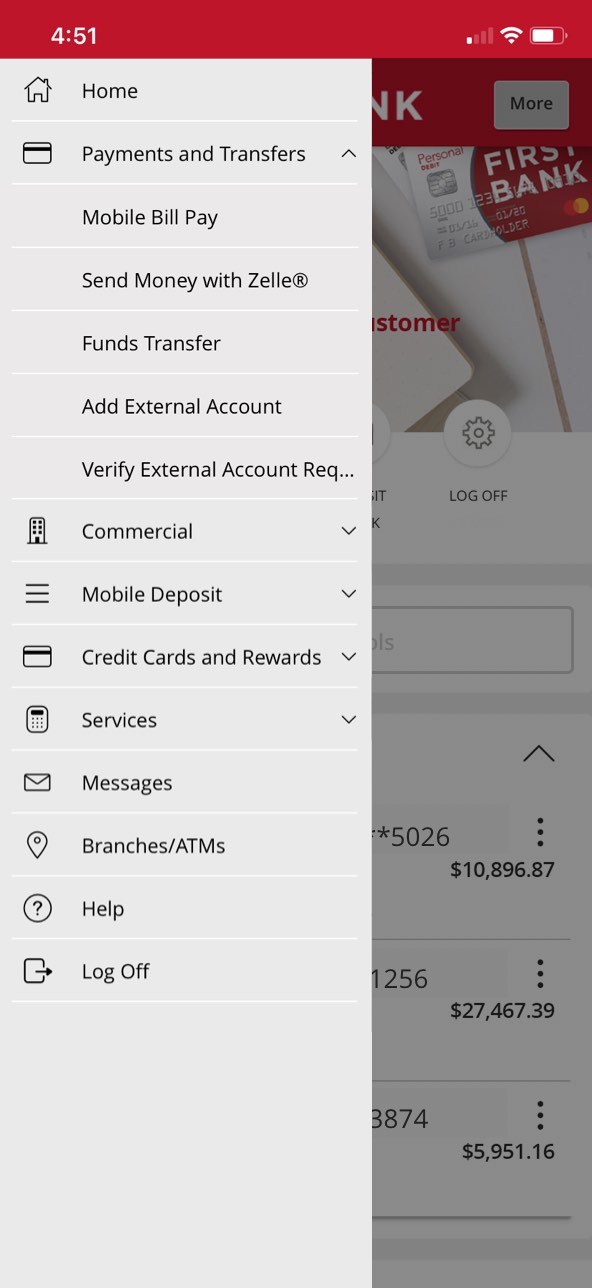### Descriptive Caption of the Mobile Banking App Screenshot:

The image is a screenshot of a mobile banking application in portrait orientation, displayed on a smartphone screen. Dominating the top of the screen is a dark red band featuring a small white text "451" in the top left corner. Adjacent to the right, there are status icons showing a very weak signal, a Wi-Fi icon, and a battery icon indicating approximately a three-quarters full charge.

On the right third of the screen, a visually subdued background image is evident. It comprises a red First Bank card with "First Bank" inscribed in white and includes a small foil hologram and a chip. This background section is overlain by a gray tint, indicating a muted lower layer where account balances are displayed. Specific account details show various balances: $10,896.87, $27,467.39, and $5,951.16, discernible by only the last four digits of the account numbers.

Dominating the left two-thirds of the screen is an off-white or pale gray menu panel stretching vertically from the top to the bottom of the display. This menu is segmented into fifteen navigable rows, each separated by thin white lines. Each row includes bold black font text and corresponding icons. The rows are arranged as follows:

1. **Home** - paired with a home icon.
2. **Payments and Transfers** - depicted with a credit card icon and clicked to expand subcategories such as mobile bill pay, send money with Zelle, funds transfer, add external account, verify external account, and a partial item marked as REQ (likely 'request').
3. **Commercial** - shown with an expandable arrow icon.
4. **Mobile Deposit** - expandable.
5. **Credit Cards and Rewards** - expandable.
6. **Services** - expandable.
7. **Messages** - with a simple black outline icon.
8. **Branches/ATMs** - with a simple black outline icon.
9. **Help** - with a simple black outline icon.
10. **Log Off** - with a simple black outline icon.

The screenshot provides a comprehensive view of both active account information and available menu options, indicative of a user navigating through First Bank's mobile application interface.